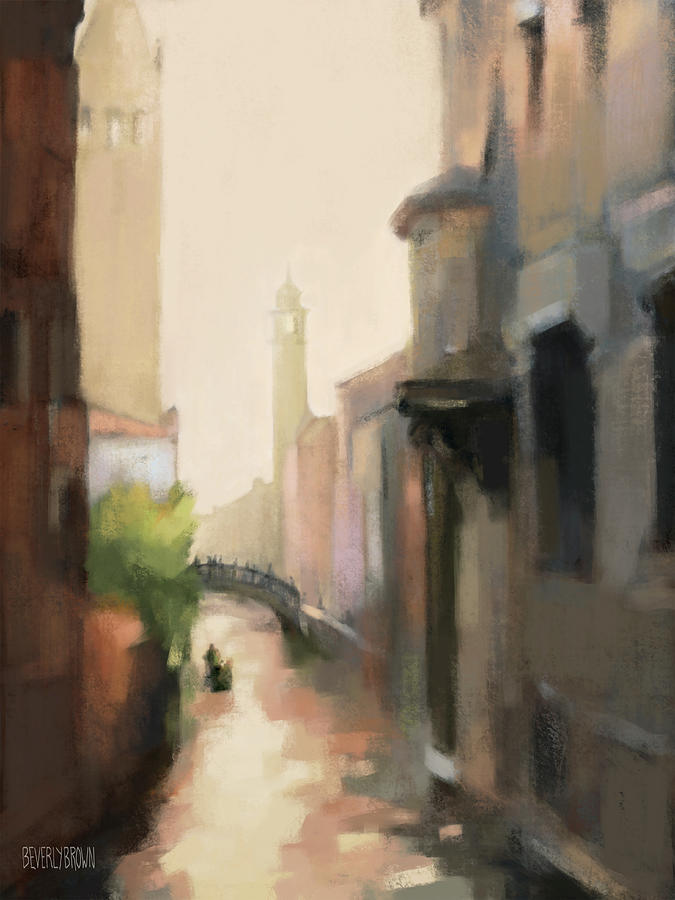This painting, likely created by Beverly Brown as indicated by her signature at the bottom, portrays a picturesque canal scene reminiscent of European river areas, possibly Venice. The canal is bordered by dark brown buildings on both sides, with additional structures and greenery, including trees, on the left. A single boat, possibly with one person, floats in the water which captures a reflective tapestry of colors, including reds and whites from the buildings and sky. An arched bridge spans the canal, with the boat positioned as though it’s about to pass beneath. In the distance, a tall tower rises, adding depth to the scene. The overall lighting suggests an outdoor setting during either sunrise or sunset, with soft beige and cream tones pervading the sky, contributing to an abstract and lightly detailed ambiance.